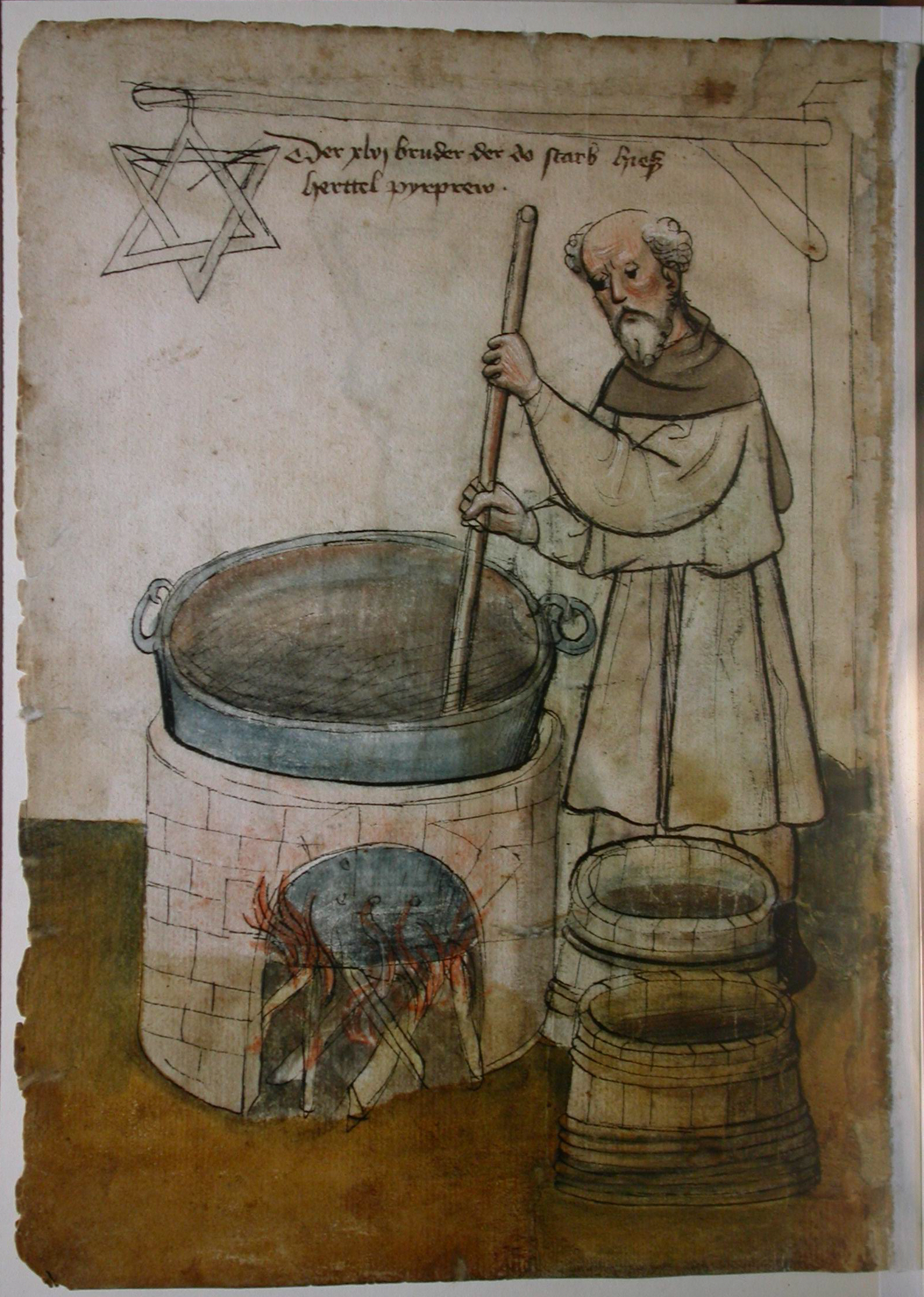This image is an old, somewhat damaged drawing portraying a scene from medieval Europe. The illustration features an elderly, bald man with white sideburns and a beard, dressed in traditional peasant attire. He is wearing a brown scarf or collar around his neck, a beige tunic that narrows at the waist and extends down to his knees, and black shoes. The man is stirring a large, metal pot placed over a fire in a brick oven or stove, using a tall wooden stick. Beside him, there are two knee-high barrels or buckets, likely filled with water. The ground beneath him appears brownish-green, possibly representing mud. Behind him, a wooden post with a horizontal arm displays a six-sided star, reminiscent of the Star of David. Some illegible cursive text, possibly in an old language like Old English or French, is inscribed at the top of the drawing. The edges of the paper show signs of wear, including tears and missing parts, giving the impression of an aged, historical piece.